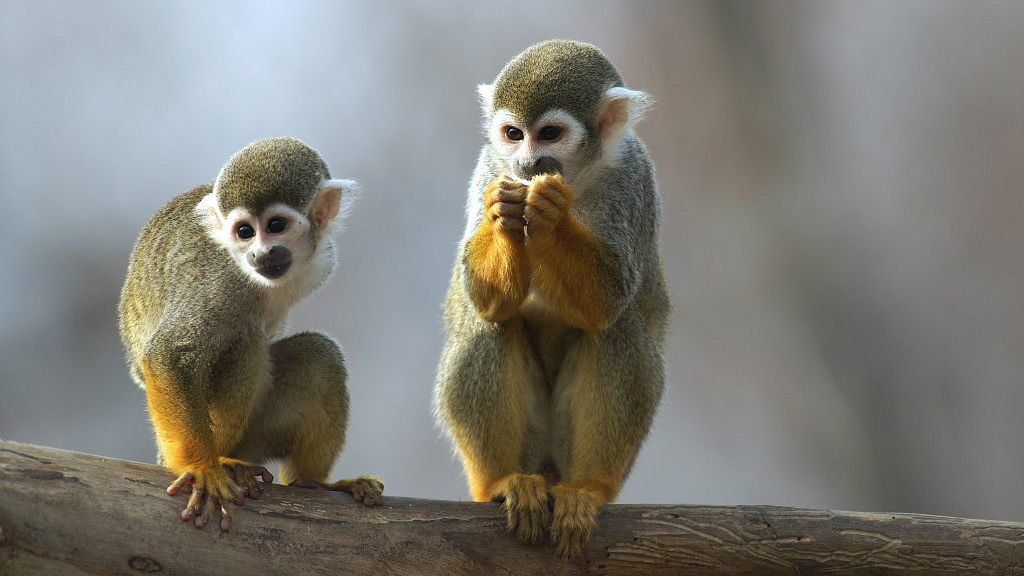In the photograph, two small monkeys are perched on a bare, sprawling branch that stretches across the bottom of the image. The backdrop is a softly blurred blend of brown, beige, and white hues, reminiscent of portrait mode on an iPhone, which adds a subtle separation from the detailed foreground. Both monkeys are looking downward, engrossed in their own world.

The monkey on the left is leaning on its right arm with a hunched back, revealing a complex mix of grayish, tannish fur with a red tint on its arms and part of its legs. Its face, surrounded by white hair, features dark, inquisitive eyes, black lips, and furry ears.

Beside it, the second monkey sits in a squatting, almost praying position with its hands clasped together near its mouth and its elbows bent, resting on its knees. It faces the viewer directly, its posture reminiscent of a contemplative squirrel. This monkey has a similarly complex fur pattern with a grayish-tannish body, highlighted with lighter brown on its hands and feet, and white fur around the eyes and ears, contrasting with its dark, expressive eyes.

The monochromatic background enhances the intricate details of their small, delicate forms and deeply intelligent eyes, making the image both captivating and serene.